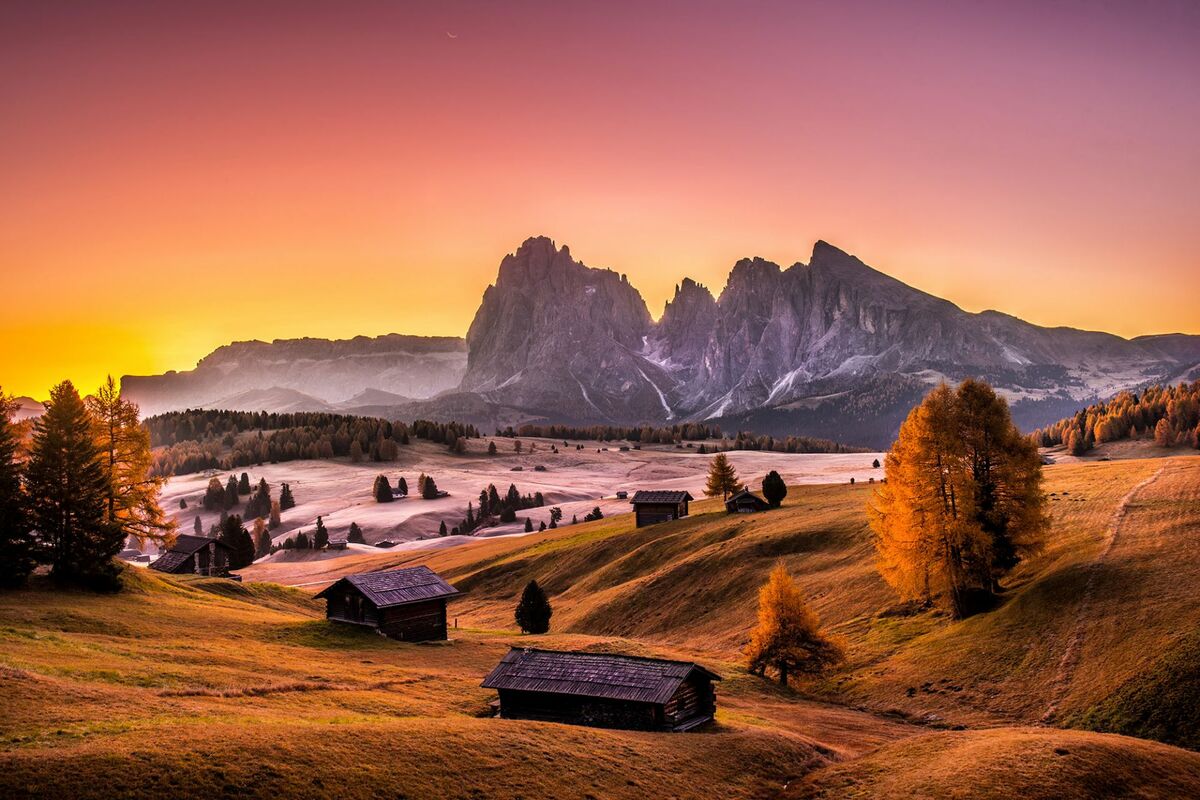This stunning image captures a picturesque landscape at dusk, characterized by a vibrant sky transitioning from deep purples at the top to pink and yellow near the horizon, where the sun has just set. Stretching across the middle of the scene are towering mountains with sharp peaks, painted in grey hues by the fading light. Below the mountains lies a sandy, whitish expanse dotted with trees. The foreground consists of rolling hills bathed in a wheat or yellowish-green tint, suggesting either sand or fall grass. Scattered throughout these hills are clusters of trees, including a notable large one to the right, accompanied by a smaller tree, and another group of trees to the left. Nestled within this idyllic landscape are several rustic, old wooden buildings, including smaller cabins and longer structures, likely made from dark, weathered wood. The scene is almost surreal in its beauty, evoking a sense of tranquility and timelessness.